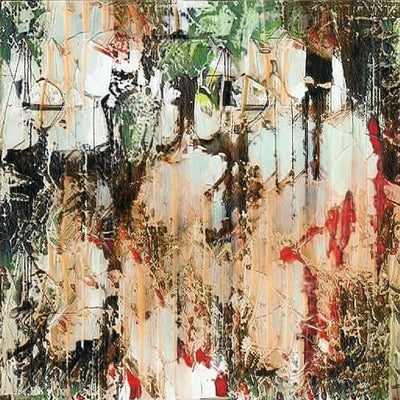The square-shaped image appears to depict an abstract piece of artwork, possibly a painting or digital illustration, characterized primarily by vertical stripes and splashes of various colors. At the top left, there are patches of black and gray, transitioning to white and brown further down. The right side starts with dark brown and black at the top, which may resemble an opening like a window. Throughout the artwork, prominent colors include various shades of green, light to dark browns, and blacks, with accents of red and pink. The background features a light, almost robin's egg blue hue, adding a subtle backdrop to the vivid colors. The bottom of the image hints at grass growing up against a slatted fence, grounding the abstract strokes in a somewhat familiar, natural setting. Overall, the piece gives an impression of stretched colors and undefined shapes, evoking a sense of nature through its organic, flowing design.